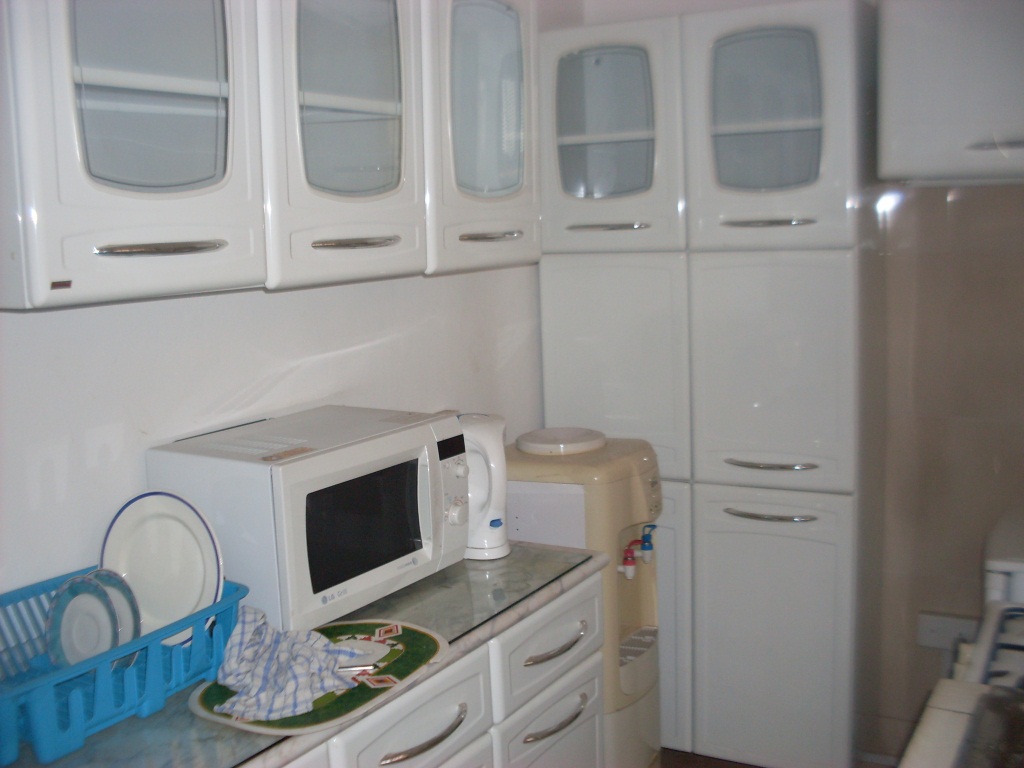The image captures a small, exceptionally clean kitchen that feels sterile and almost office-like, primarily defined by its unique shelving and white appliances. Dominating the top third of the image, there are white, plastic-like shelves with a large, transparent plastic window front and a silver strip near the bottom. Within this window, several white shelves are visible. Below this setup, you'll find rows of white shelves along the left wall and spilling over to the adjacent corner. To the right, there are more white shelves featuring silver handles.

In the top right corner of the photo, there is a plain white shelf with a silver strap underneath. The lower half of the kitchen presents two rows of long white shelves without windows, each with different handle placements. Below these shelves and set against a white wall is an older-looking, white microwave with a black viewing window and two knobs of different sizes below a digital clock.

On the countertop next to the microwave sits a dish strainer containing two small saucers with blue rims and a larger plate with a dark blue trim. A green mat lies on the marbled counter with a blue and white rag placed on it. Beneath this setup, the front of the countertop reveals drawers and a large cupboard door, all adorned with big silver handlebars.

In the center-left of the kitchen, there's a water dispenser for hot and cold water, typically found in offices, complete with red and blue handles. To its right, an electric kettle is perched on the counter. The kitchen also houses other appliances, possibly an oven or a hob, and a refrigerator in the corner stands out due to its tan-beige color, breaking the predominant white theme of the space. This spotless kitchen nook area is designed to fit one, or perhaps two people at most, adding to its cozy, compact feeling.